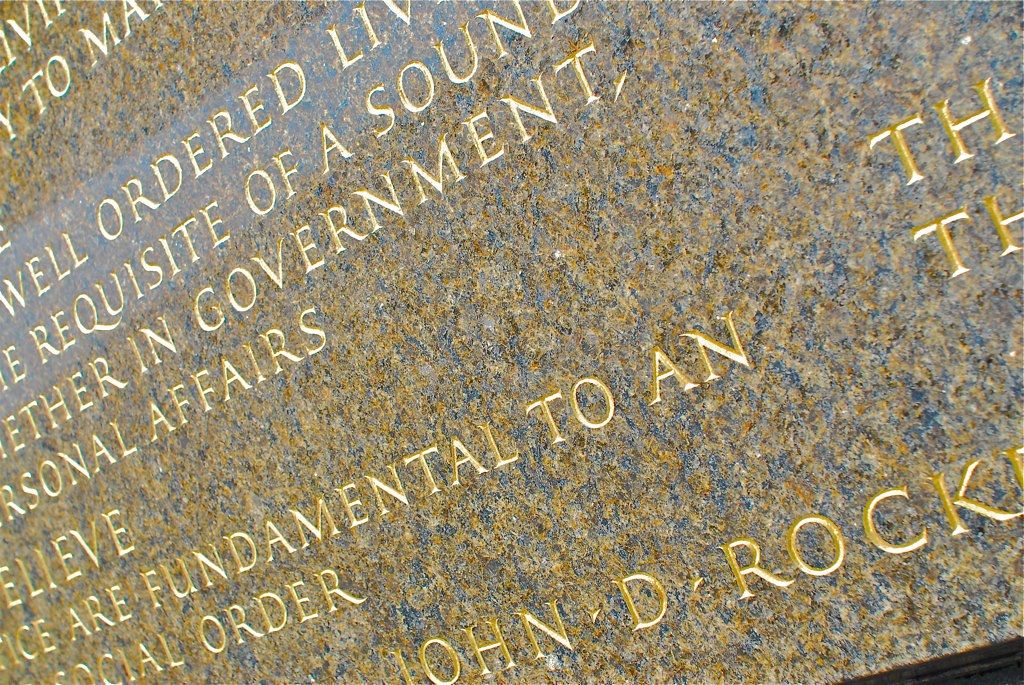This image is a close-up of a monument made from smooth marble, characterized by a striking blend of blue, beige, and tan colors. The marble slab is tilted to the left, and prominent, well-ordered gold engravings embellish its surface. The text, written in capital letters and in English, spans diagonally from the bottom left to the top right, though many words are partially cut off. The legible segments of the inscription include "the requisite of a sound," followed by "in government or personal affairs," ending with "fundamental to a social order." At the bottom of the slab, the name "John D. Rock" is visibly inscribed, likely referencing John D. Rockefeller. The detailed gold lettering adds a distinguished touch to the monumental stone, suggesting a significant memorial.